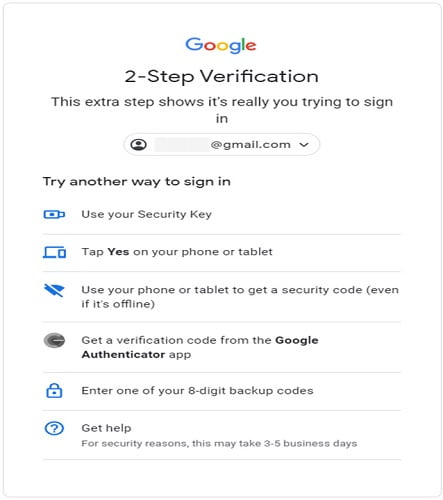**Detailed Caption:**

The image is a screen capture of a Google two-step verification page. At the top, the familiar Google logo is prominently displayed, featuring the characteristic blue, red, yellow, and green colors. Directly beneath the logo, the text reads "Two-step verification," indicating it is an authentication step to enhance security.

Below this header, there's a message stating, "This extra step shows it's really you trying to sign in," followed by an email address placeholder "[name]@gmail.com," although the actual name is obscured. Underneath the email address, there are several options for verifying the user's identity, each accompanied by a unique icon for better visualization:

1. **Try another way to sign in:** An option suggesting alternatives if the user can't proceed with the current method.
   
2. **Use your security key:** This option features an icon that appears to depict either a keyboard or camera next to it, indicating a security device.

3. **Tap Yes on your phone or tablet:** Here, a blue icon resembling a laptop or smartphone instructs the user to confirm their sign-in on another device.

4. **Use your phone or tablet to get a security code even if it's offline:** This illustrates using a mobile device to receive a code, facilitated by a phone/tablet icon.

5. **Get a verification code from the Google Authenticator app:** This option suggests using the Google Authenticator app.

6. **Enter one of your 8-digit backup codes:** Depicted by a lock icon, this method allows the input of a pre-generated backup code for verification.

7. **Get help:** Accompanied by a question mark icon, this speaks to further assistance options, where it states for security reasons, the process may take three to five business days.

Each of these steps emphasizes Google's layered approach to maintaining account security and ensuring that only the legitimate user can gain access.

This well-structured layout provides multiple methods to complete the verification process, thereby accommodating different user needs and scenarios.